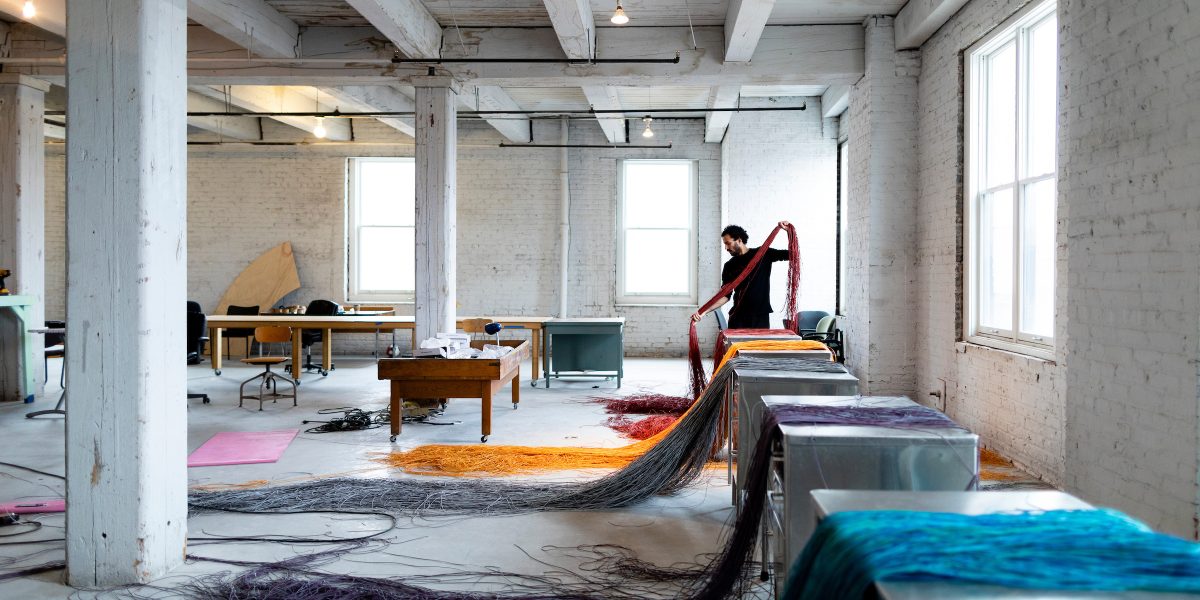In this image, we see the interior of a bright, spacious workspace with an industrial vibe. The walls are whitewashed brick, giving a clean, airy feel to the room, which is further accentuated by the natural light streaming in through several windows—one on the right and two at the back. White stone columns and painted beams support the ceiling, adding to the structural aesthetics of the space.

Aligning the right-hand side, there is a series of five tables covered with different strands or fabrics, each dyed in distinct colors: blue, purple, gray, orange, and red. The fabrics appear to drape elegantly over the edges of the tables and trail onto the floor. Amidst this setup, a man dressed entirely in black, with dark curly hair and a beard, stands prominently, holding one of the red strands.

The workspace is equipped with several surfaces, some metallic and others wooden, indicating a busy, creative environment. To one side, a few wooden desks are arranged, suggesting areas for more detailed or administrative tasks. A glimpse of a pink yoga mat on the floor hints at a touch of relaxation amidst the bustling activity. The overall aesthetic combines functionality with a touch of artistry, making it a unique and inspiring place to work.